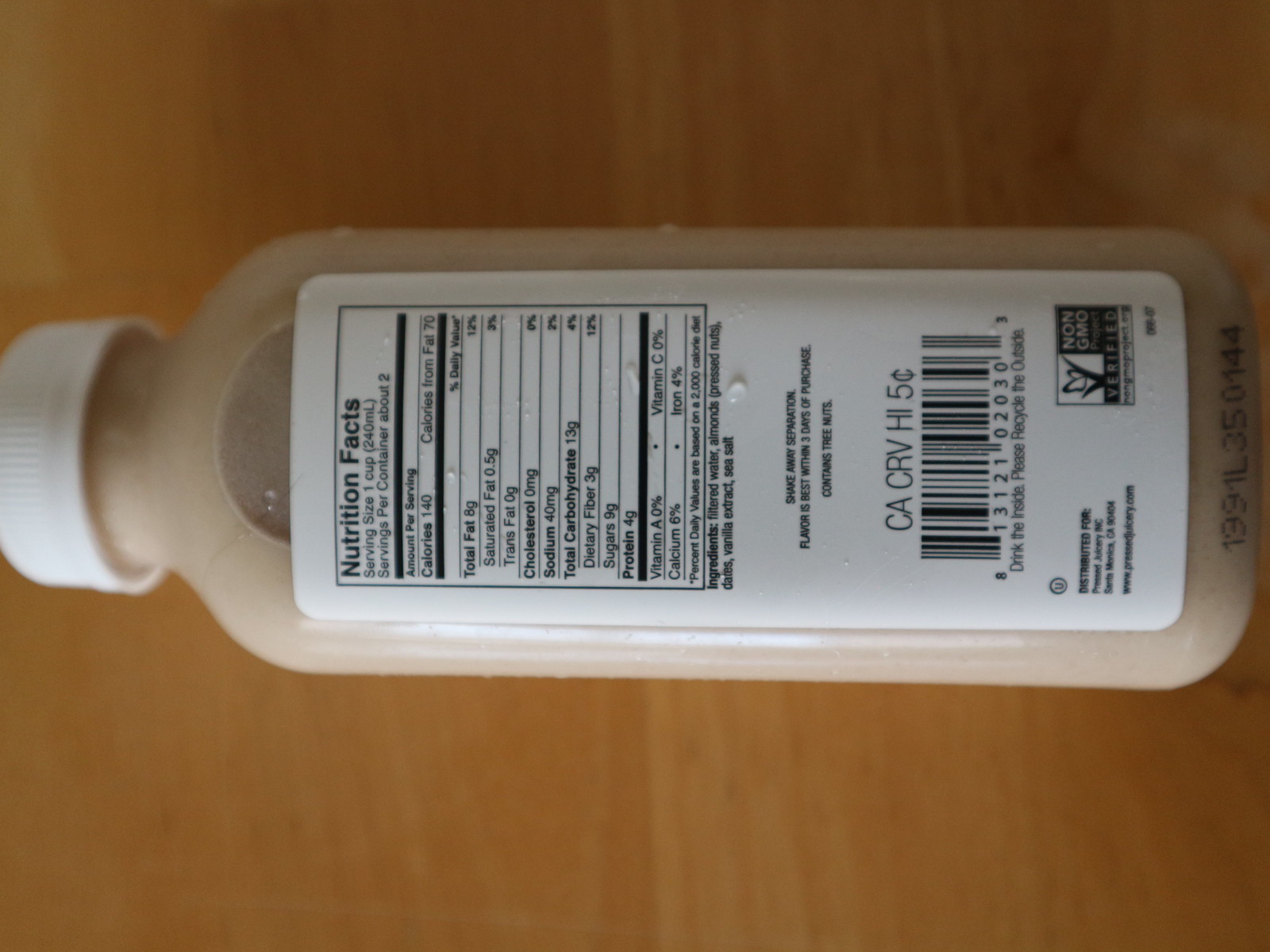The photograph captures an indoor scene featuring a close-up of a bottle placed on a wooden surface. The light tan wooden surface, adorned with subtle wood grain patterns, contrasts gently with the clear bottle. The bottle, viewed from the back, reveals a label with nutrition facts and a white cap sealing its contents. The light brown liquid inside the bottle suggests it might be some kind of flavored almond milk or a similar beverage. The label details list filtered water, almonds, vanilla extract, sea salt, and pressed nuts as the main ingredients. Nutritional information indicates one cup per serving, with two servings in total, and 140 calories per serving. A barcode, additional label information, and a serial number are printed beneath the nutrition facts, completing the detailed depiction of the bottle.